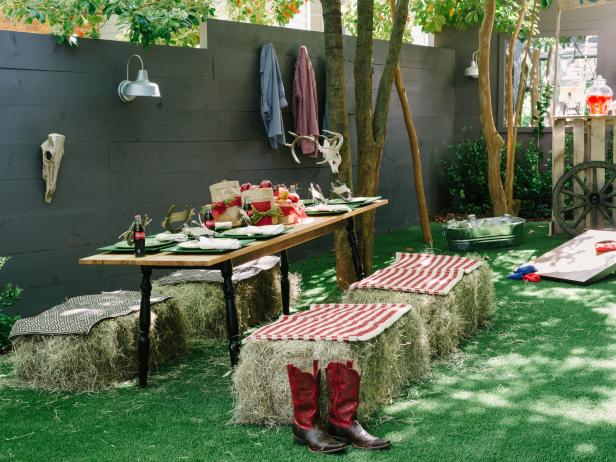The image depicts an outdoor scene, likely set in someone's backyard, designed with a farm-themed party ambiance. Dominating the background is a long, rectangular, dark gray cement wall decorated with a mounted light and a skull, possibly from a cow. Clustered around the base of the wall are two shirts – one blue and one red or pink – hanging casually. To the right of the scene, two interconnected trees branch out with lush green leaves, creating a natural canopy above.

Below the wall, the ground is covered in green grass. Central to the setup is a rustic wooden table with black spindle legs, which is laden with a charming arrangement of party essentials. The table is set for approximately eight people, featuring white plates on green platters, a basket of apples, a bottle of Coke, and a central beige and red centerpiece with green bows.

In front of the table lie four bales of hay, two on each side, draped with red and white cloths, presumably serving as seating. The hay seating arrangement is complemented by a pair of red and brown cowboy boots placed prominently in the middle. The overall setting reflects a relaxed, festive atmosphere basking under the sun.